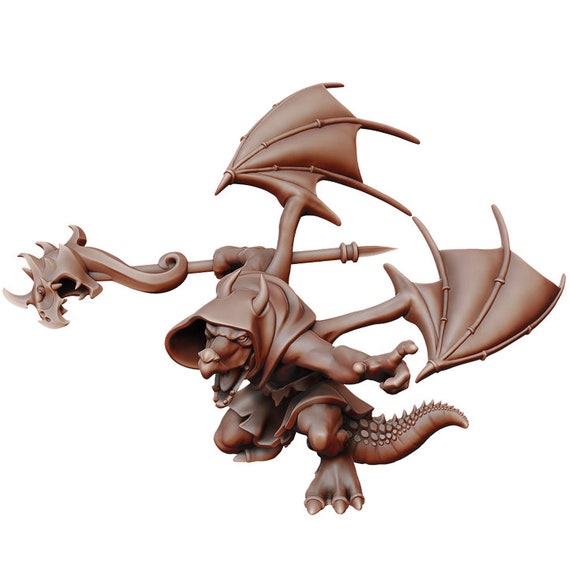The image depicts a detailed sculpted figurine of a menacing creature that appears to be a goblin-dragon hybrid, rendered in a rich, reddish-brown color, reminiscent of milk chocolate. The figurine, which showcases characteristics of both a dragon and a lizard, has a scaly, spined tail and muscular, humanoid arms that extend outward. In its right hand, it clutches a staff topped with a horned, dragon-like head and a spike at the back.

The creature features distinct red eyes set in a lizard-like snout and is adorned in a hooded cloak with holes for its protruding horns. The cloak is belted at the waist, giving it a skirt-like appearance around the thighs. The figurine's feet are wide and webbed, ending in three clawed toes, while its bat-like wings—complete with spiky, bony points—are spread wide behind it.

The creature has human-like, albeit slightly stubby, fingers and appears to be snarling or screaming with its mouth open, enhancing its villainous, fantasy-game aesthetic. The detailed scales run along its back, contributing to the figure's reptilian texture. This intricately designed piece is showcased against a plain white background, emphasizing its vivid three-dimensional form and making it reminiscent of a digital rendering from a fantasy game or a vinyl/metal figurine.